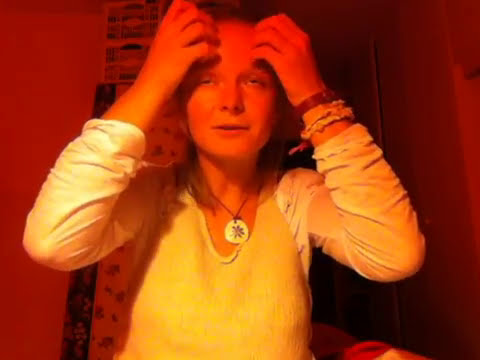The photograph depicts a woman seated in a red-lit room, facing the camera. The intense red tint of the lighting gives both her face and the room's walls a reddish hue. She appears either exhausted or startled, with her mouth slightly open and her half-closed eyes conveying a sense of weariness or disbelief. Her hands are pressed against her forehead, fingers curled as if attempting to part her hair or alleviate a headache. She is dressed in a white shirt that looks particularly soft and comfortable, and around her neck, she wears a black cord necklace with a sizable circular pendant, featuring a dark blue floral pattern on a white background. On her left wrist, she sports an assortment of bracelets: one red rubber or plastic bracelet, one rough, ruffled fabric bracelet, and possibly a leather bracelet or a watch worn backwards. In the background, the room's walls glow red due to the lighting, and an open door is visible on the right side of the scene.